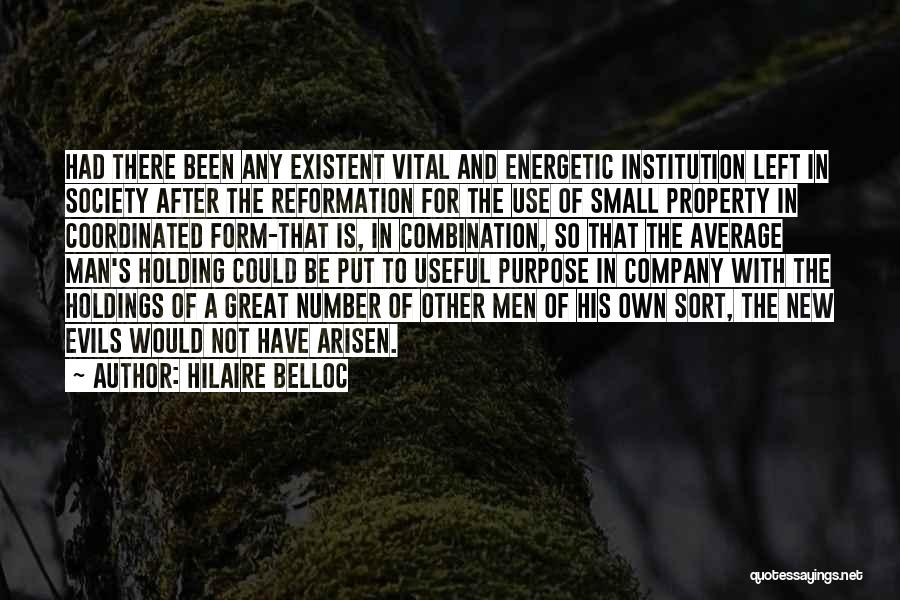The image features a detailed quote from the author Hilaire Belloc, printed in black capital letters on a white background, superimposed over a dark, moss-covered tree branch. The lush, green moss extends across the thick trunk and smaller branches, some of which are plain brown. The scene is set against a frosty, white ground with pieces of white frost scattered about, enhancing the stark contrast between the dark, natural elements and the crisp text overlay. The quote reads: "Had there been any existing vital energetic institution left in society after the Reformation for the use of small property in coordinated form, that is, in combination so that the average man's holding could be put to useful purpose in company with the holdings of a great number of other men of his own sort, the new evils would not have arisen." The author's name, Hilaire Belloc, appears beneath the quote, preceded by a tilde. At the bottom right of the image, the website address quotesayings.net is printed in small white text.